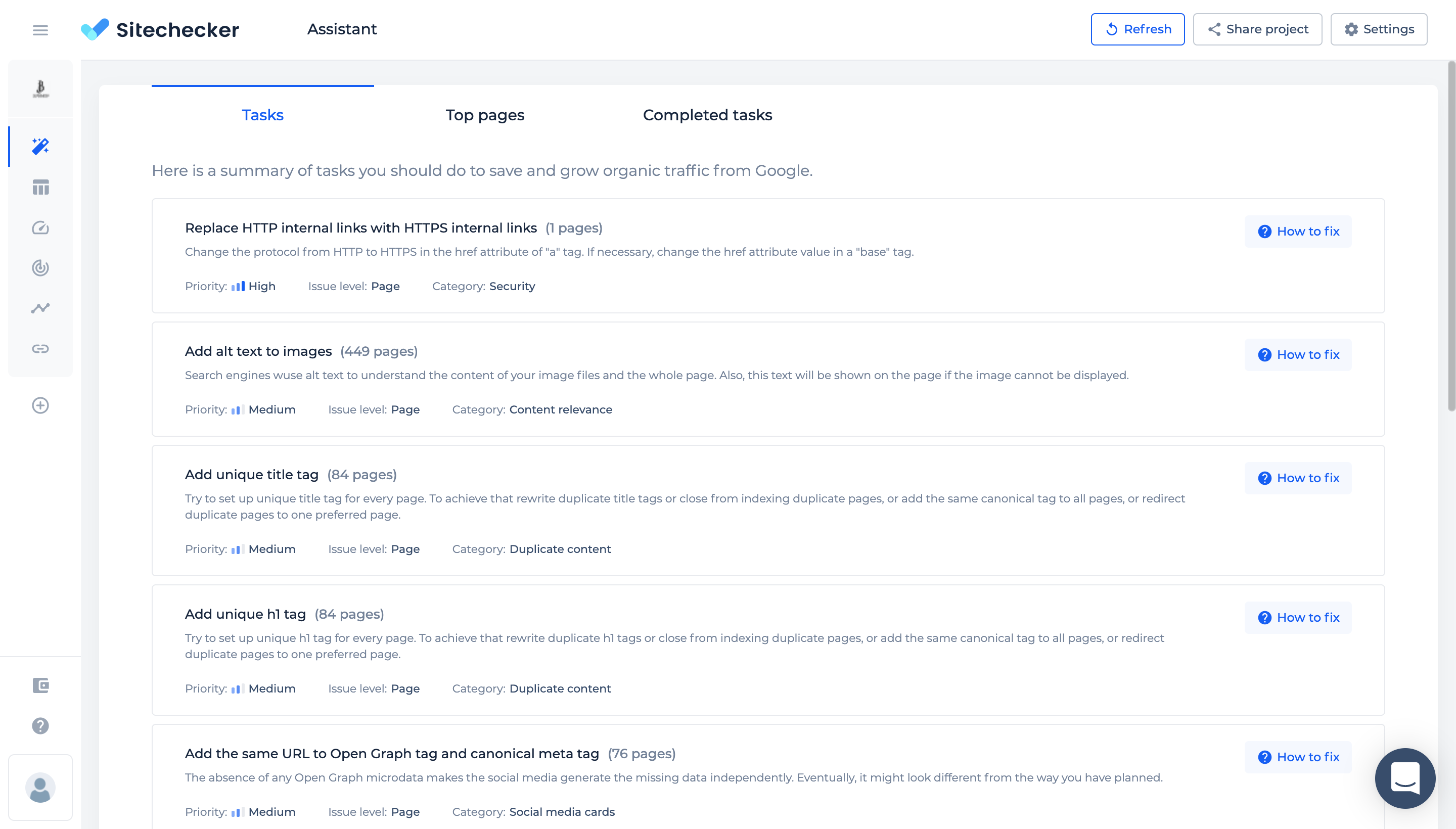The image showcases a webpage from the Sitechecker tool, specifically the 'Assistant' section. On the right side of the interface, there are three action buttons: 'Refresh,' 'Share Project,' and 'Settings.' The main content area contains three tabs: 'Tasks,' 'Top Pages,' and 'Completed Tasks,' with the 'Tasks' tab currently selected. 

Under the 'Tasks' tab, a summary lists steps to enhance and grow organic traffic from Google, including instructions such as:
1. Replace HTTP internal links with HTTPS internal links.
2. Add alt text to images.
3. Add unique title tags.
4. Add unique H1 tags.
5. Add the same URL to both the Open Graph tag and the canonical meta tag.

On the left side, there are ten icons, with at least one recognizable as a plus mark, although the others are unidentified. At the bottom of the interface, there is a user sign-in option. The clean layout and detailed recommendations provide users with a clear roadmap for optimizing their website’s SEO.